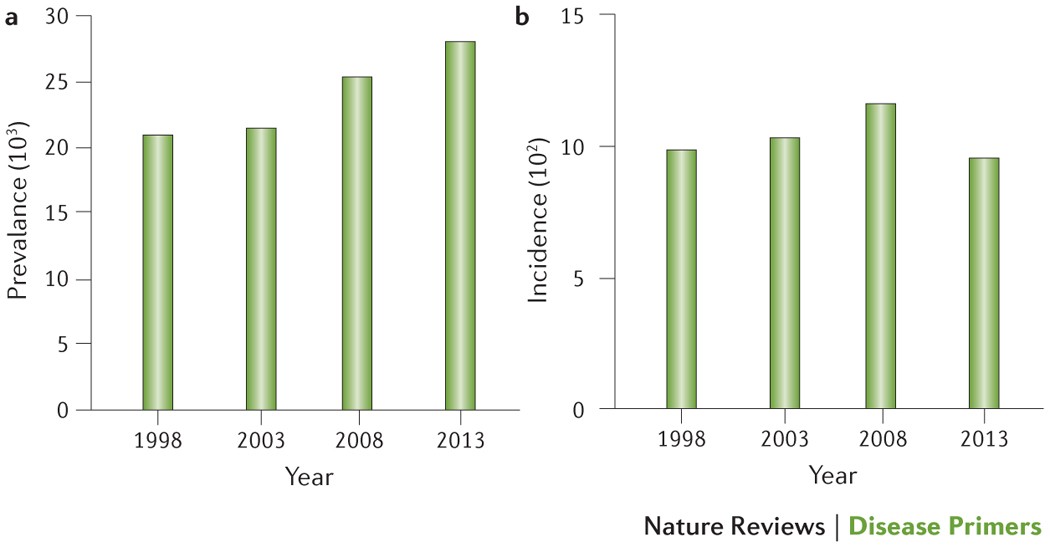The image displays two side-by-side bar charts labeled "Nature Reviews Disease Primers." The left chart, Chart A, shows prevalence with the y-axis labeled "Prevalence (10^3)" and the x-axis marked by the years 1998, 2003, 2008, and 2013. The prevalence scale ranges from 10 to 30, illustrating an increasing trend across the indicated years. On the right, Chart B depicts incidence with the y-axis labeled "Incidence (10^2)" and the same years on the x-axis. The incidence scale ranges from 0 to 15, with all years hovering around a value of 10. Both bar charts use shaded green cylinders to represent data values.